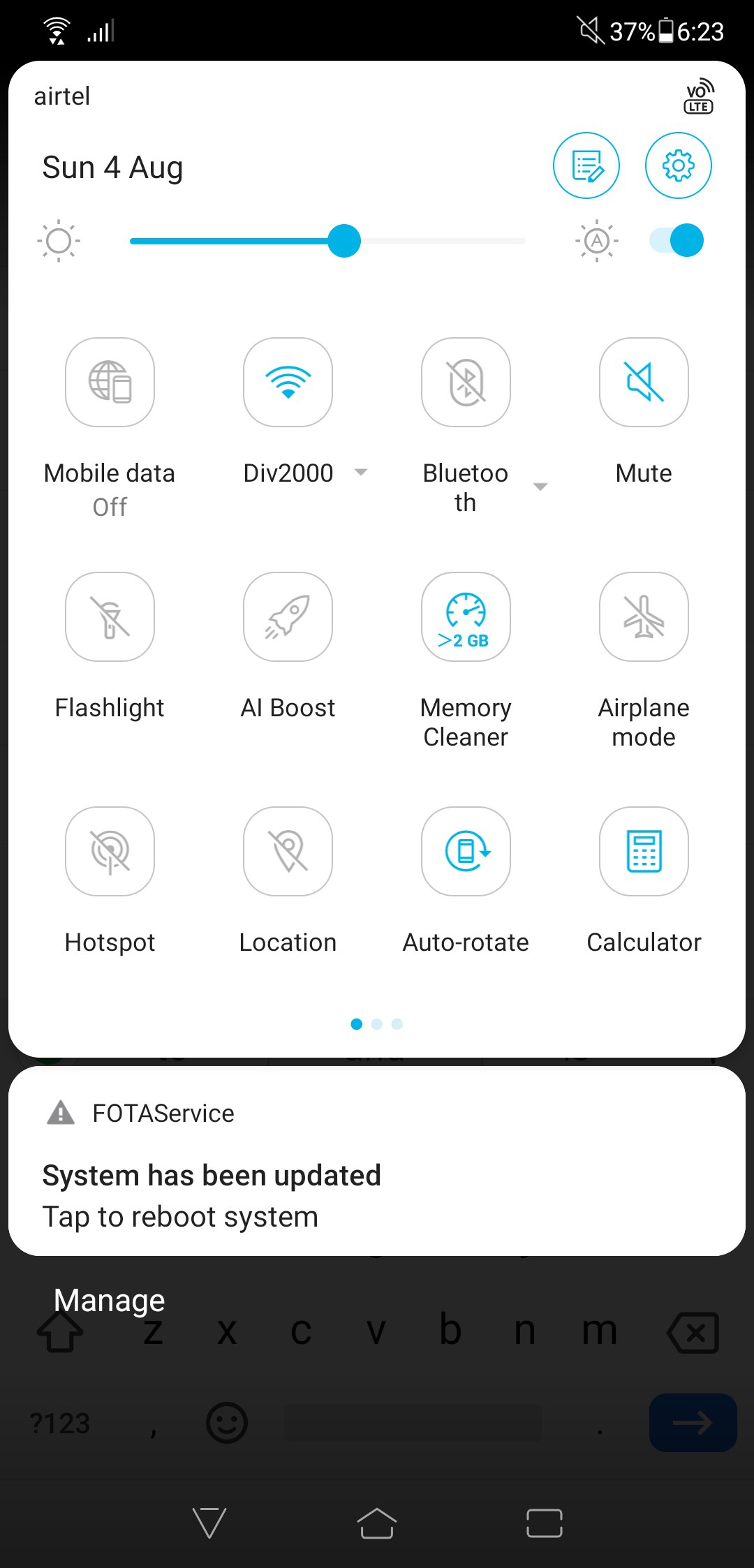The image depicts a screenshot from an Android mobile device, offering a detailed overview of its status and settings:

1. **Status Bar (Top Left to Right):**
   - **Wi-Fi:** Indicator shows full signal strength.
   - **Cellular Signal:** Four bars present.
   - **Silent Mode:** Phone is on mute.
   - **Battery:** 37% remaining.
   - **Time:** 6:23.
   - **Date and Provider:** Sunday, 4 August, connected via Airtel.

2. **Quick Settings Panel:**
   - **Icons:**
     - **Pencil:** Editable mode toggled on.
     - **Cogwheel:** Settings toggled on.
   - **Brightness:** Approximately 50%, with automatic brightness enabled.
   - **Mobile Data:** Disabled (represented by a globe and cell phone icon).
   - **Wi-Fi:** Enabled and connected to network "DIV2000".
   - **Bluetooth:** Disabled.
   - **Silent Mode:** Enabled.
   - **Flashlight:** Disabled.
   - **AI Boost:** Enabled (icon of a rocket ship).
   - **Memory Cleaner:** Enabled, shows less than 2GB available (icon of a fuel gauge).
   - **Airplane Mode:** Disabled.
   - **Hotspot:** Hotspot feature appears inactive.
   - **Location Services:** Disabled.
   - **Auto Rotate:** Enabled (icon of a phone with a circular arrow around it).
   - **Calculator:** Enabled, indicated by a blue calculator icon.

3. **Notifications:**
   - **FOTA Service Notification:** 
     - **Content:** System updated, tap to reboot.
     - **Options:** "Manage" button available.
   - **Navigation Buttons:**
     - **Arrow (Back):**
     - **Home (House):**
     - **Recent Apps (Square):**

The screenshot comprehensively displays the device's settings and status, providing insights into the connectivity, system updates, and various toggled features. This includes details specific to the phone's current states, such as connectivity options, system brightness, and active applications, highlighting the concise environment of the device's operational mode at that moment.